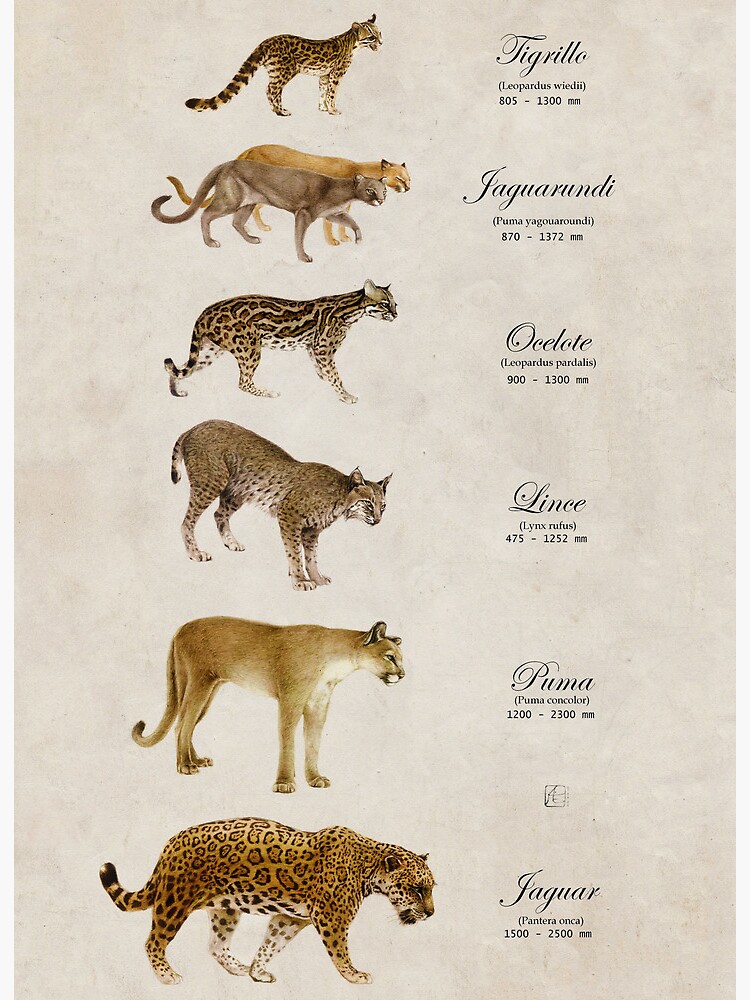The image is a detailed painting depicting six wild cats arranged vertically from top to bottom against a light gray background, with each cat's name inscribed to the right accompanied by additional information. At the top is the Tigrillo, a small feline resembling a leopard, characterized by its black prints on an orange and white body, along with a long tail. Below the Tigrillo are two Jaguarundis, presented in a pair with one gray and one orange cat, both solid tan in color and noted for pacing side by side. The central position features an Ocelot, which has an orange body with distinct brown and black patterns and more random spots compared to a leopard. Below the Ocelot is the Lynx, similar in size but lighter in shade, adorned with random spots and notable for its very short tail. Next is the Puma, also referred to as a mountain lion, tan-colored with a white chest and a long tail. At the bottom is the Jaguar, the largest of all, distinguished by its extensive spots and tail that ends in a black bush.